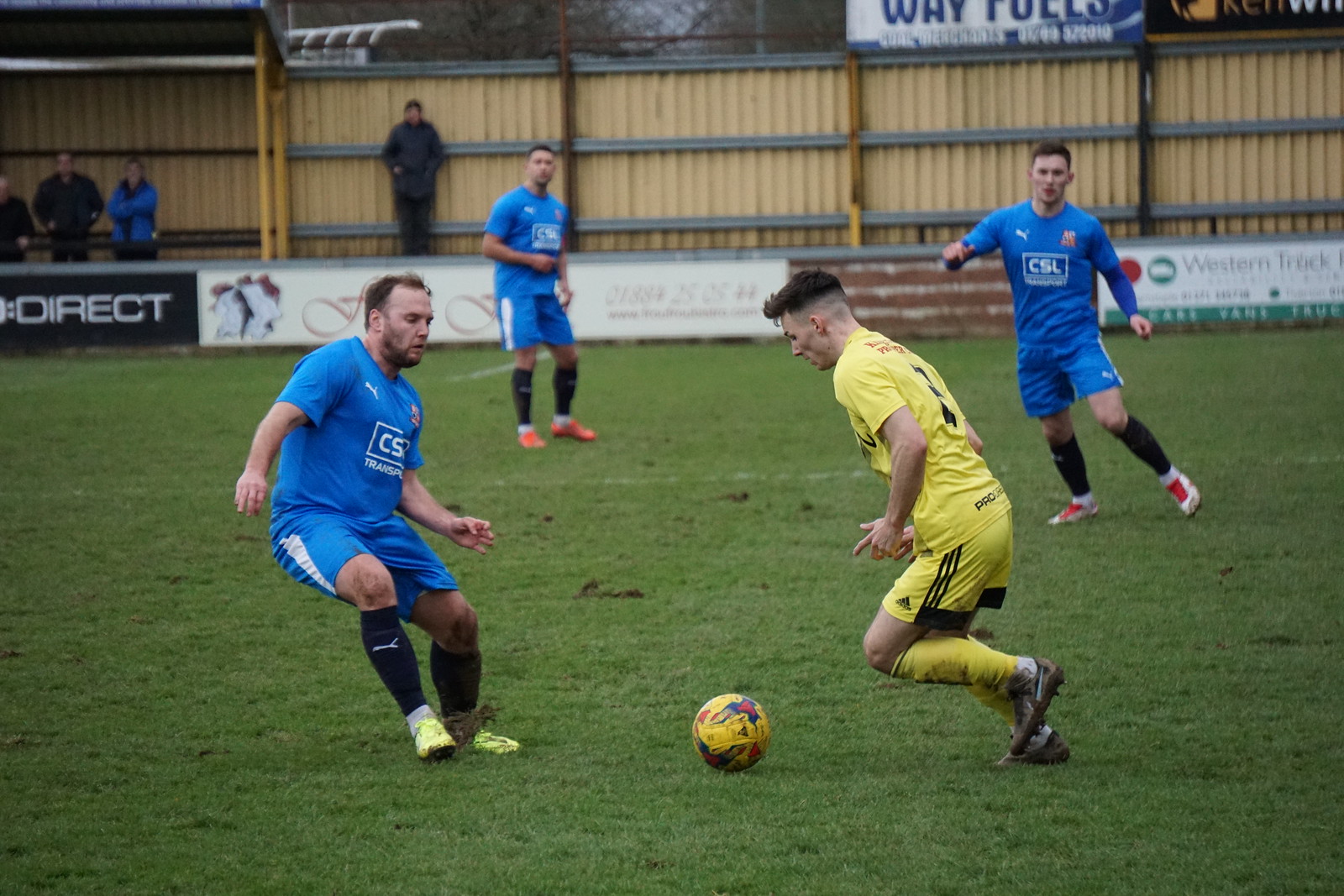In this detailed image of a soccer game in action, we see four players prominently featured on a grass field. The field has several patches where the grass is worn thin. Three of the players are dressed in matching blue uniforms: blue shirts with white lettering on the chest, blue shorts with white stripes, and blue socks. Their cleats vary in color, with one wearing yellow, another orange, and the third in red and white cleats. Each player in blue is equipped with leg protectors. There is a notable interaction in the foreground where one of the men in blue is playing defense against a player in a yellow uniform, who is on offense and actively kicking a yellow soccer ball. The player in yellow sports a complete yellow kit: yellow shirt with short sleeves, yellow shorts adorned with three black stripes and an Adidas logo, yellow knee socks, and black cleats that appear very muddy. Behind a brown fence encircling the field, several spectators are visible, some donning jackets while standing and watching the match intently. Additionally, there are individuals seated on a bench in the upper left corner and various advertisement signs on display around the field.